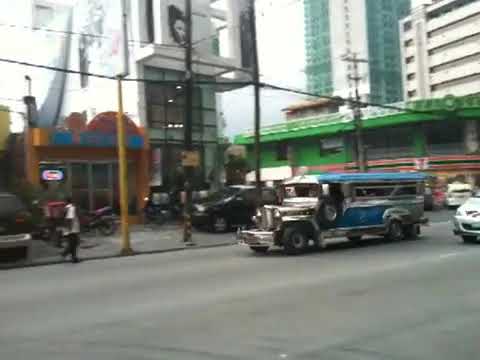This daytime outdoor photograph, though blurry and of low quality, distinctly captures a lively street scene in Manila, Philippines. Dominating the foreground is a distinctive jeepney, known for its origins as a decommissioned U.S. military vehicle repurposed into a hybrid between a truck and a bus. This particular jeepney has a shiny silver metal front, resembling a school bus or semi-truck cab, and a flat blue roof extending to the bus-like rear. The spare tire is oddly situated where one might expect the driver's side door to be. Surrounding the jeepney, the paved roadway is devoid of markings and is a light gray color.

To the left, there is a short orange building adorned with blue print, though the text remains unreadable. Directly behind the jeepney sits a 7-Eleven store, above which rises a green building. Further into the background, a combination of tall buildings, potential parking structures, and skyscrapers dominate the skyline. The right side of the scene features another prominent green building. Additionally, the scene includes several street lamps of varying colors, including yellow and black, and power lines crisscrossing in the background. A man can be seen walking on a walkway behind the jeepney, contributing to the dynamic urban atmosphere of the photograph.